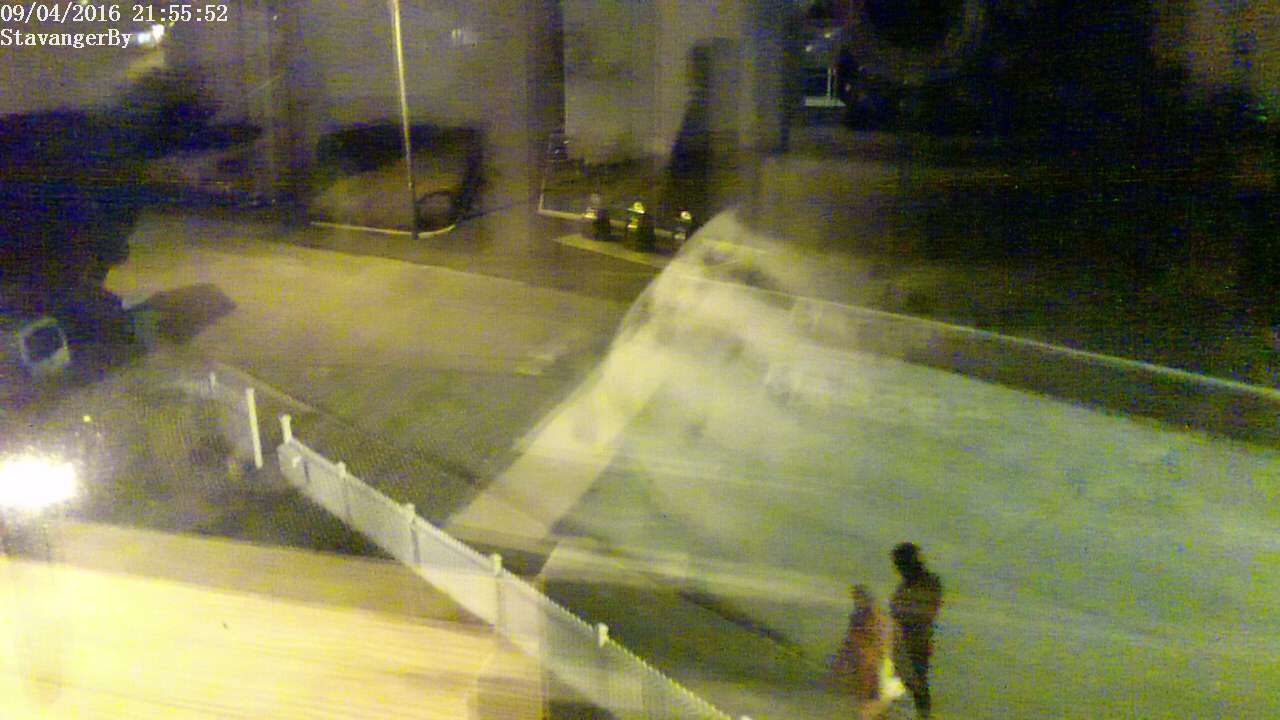A man and a woman walk side by side down a wide concrete pathway beneath the night sky. The man, dressed entirely in black, strides to the right, while the woman, clad in brown attire, walks on his left. To their left, a white fence runs parallel to their path, while towering buildings with glass windows dominate the right side of the scene. Through the windows, faint silhouettes of objects are just visible. A mysterious large dark shape looms indistinctly farther down the street, partly concealed around a corner. The area is softly illuminated by a couple of streetlights, casting a bright light on the left side and creating gentle reflections in the center.